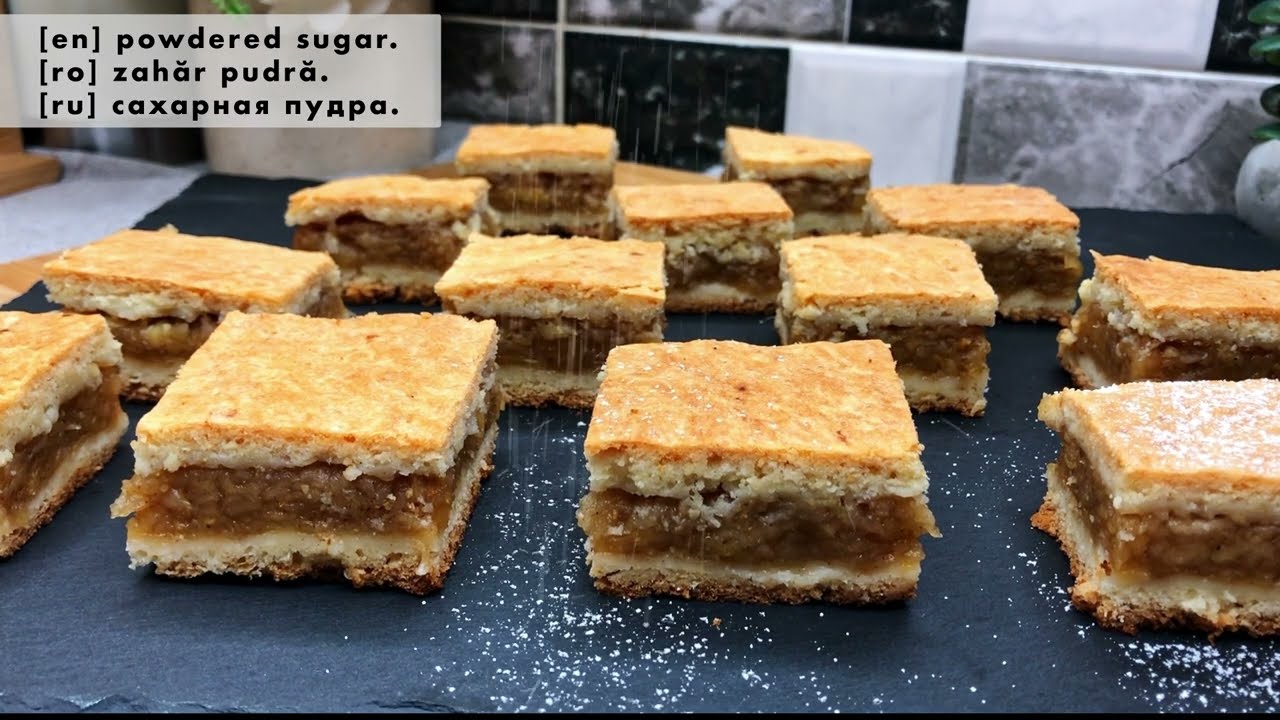The image shows an array of pastries neatly arranged in a triangular pattern on a dark blue or gray platform, which could be a table or tray. These pastries feature a flaky, layered structure with a darker brown bottom layer, topped with a slightly lighter brown upper layer. Within these layers, there is a gooey, custard-like filling that resembles chopped apples or apple butter. Some pastries are sprinkled with powdered sugar. The backdrop includes a wall decorated with black, white, and gray tiles. A rectangular box in the image reads "powdered sugar" in multiple languages: English (EN), Romanian (RO, Zaharpudra), and Russian (RU, Caxifar Nayapa). The picture is taken from a low angle, almost level with the pastries, emphasizing the texture and details of the treats.